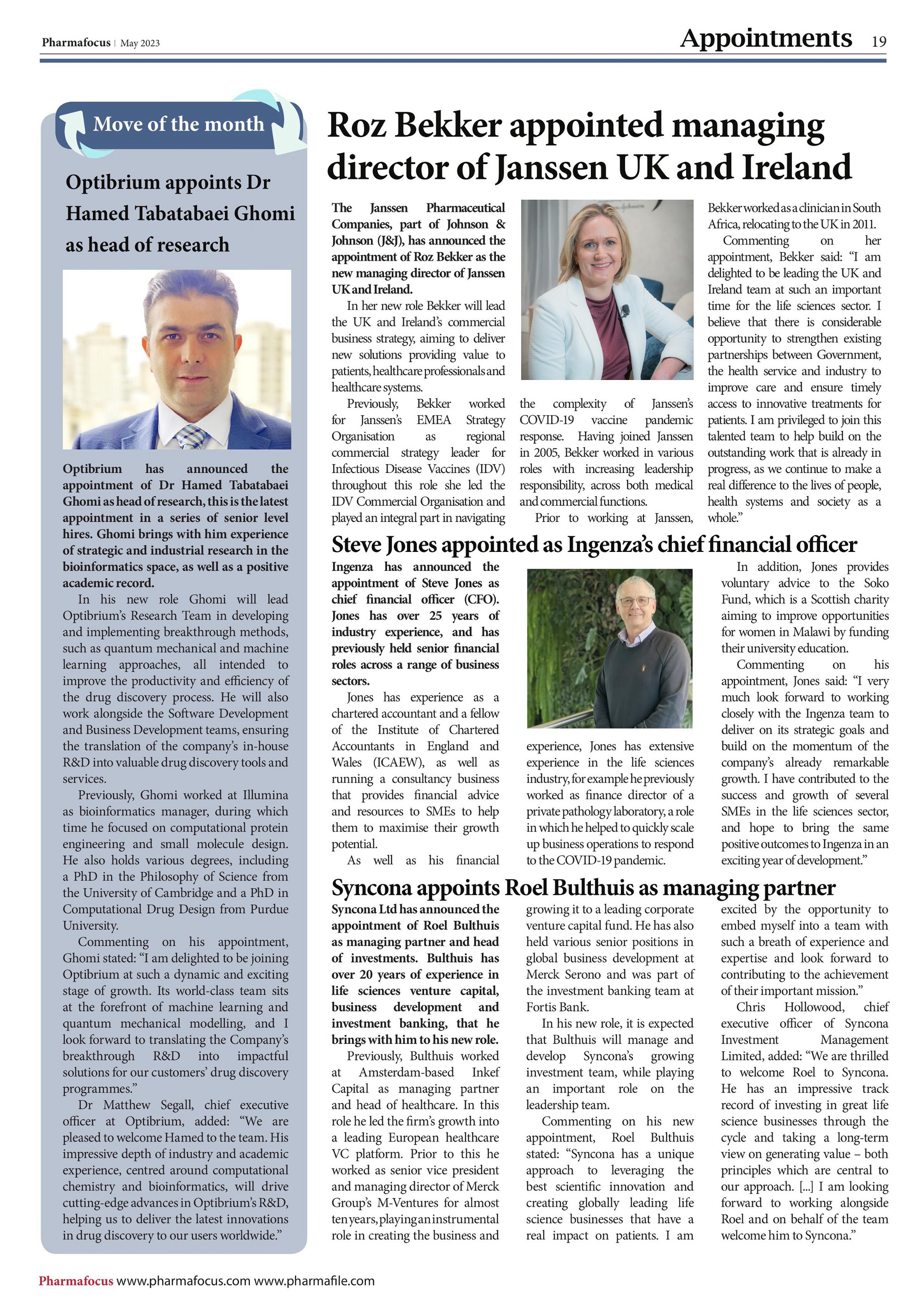This detailed caption concisely describes the contents and layout of the "PharmaFocus" page from May 2023:

---

This page from the May 2023 issue of PharmaFocus features important appointments in the pharmaceutical industry. The top-left corner displays the PharmaFocus logo in black, alongside the date "May 2023." On the top-right corner, the word “Appointments” is prominently printed in black with the page number "19" next to it, indicating this is page 19.

The left-hand column is shaded in a grayish-blue hue and is titled "Move of the Month." It highlights the appointment of Dr. Hamid Tabaki Gomi as Head of Research at Optibrium.

The rest of the page is set against a white background and comprises three different appointment reports:
1. **Roz Becker Appointed Managing Director of Janssen UK and Ireland**: This article includes a small square photo of Roz Becker, a white female with blonde hair.
2. **Steve Jones Appointed as INGESA's Chief Financial Officer**: Accompanying this article is a small photo of Steve Jones, an older man with some gray hair, wearing glasses, a grayish-black sweater, and a long-sleeve collared shirt underneath.
3. **Syncona Appoints Roel Bothis as Managing Partner**: This article does not include a photo of Roel Bothis.

At the bottom-left corner, the website URLs www.pharmafocus.com and www.pharmafile.com are listed in black text next to the word "PharmaFocus" in red.